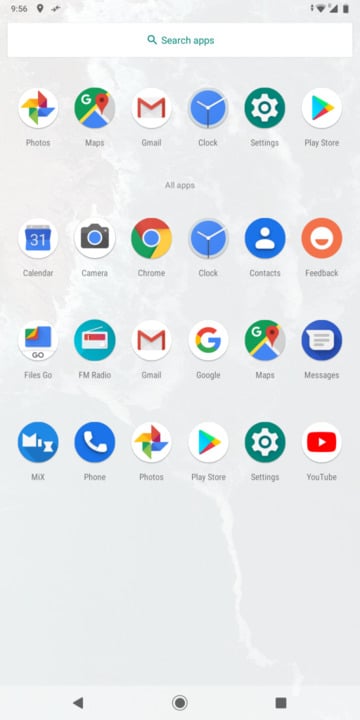This is a detailed screenshot from a mobile phone displaying the home screen. The background features a minimalist gray design with a white curving pattern. At the top of the screen, the time is prominently displayed as 9:56. Below the time, there is a white search bar with the text "Search apps."

The screen is populated with app icons, arranged in a grid format from left to right and top to bottom. The sequence of apps is as follows: Photos, Maps, Gmail, Clock, Settings, Play Store, Calendar, Camera, Chrome, Clock (repeated), Contacts, Feedback, Files Go, FM Radio, Gmail (repeated), Google, Maps (repeated), Messages, Mix, Phone, Photos (repeated), Play Store (repeated), Settings (repeated), and YouTube.

At the bottom of the screen, there are three navigation buttons: a black arrow pointing to the left (back button), a black circle (home button), and a black square (recent apps button).

This image has a portrait orientation, making it much taller than it is wide. There are no photographic elements or visual representations of people, animals, plants, flowers, trees, or automobiles on this cell phone screenshot. It strictly displays the digital interface and app icons.